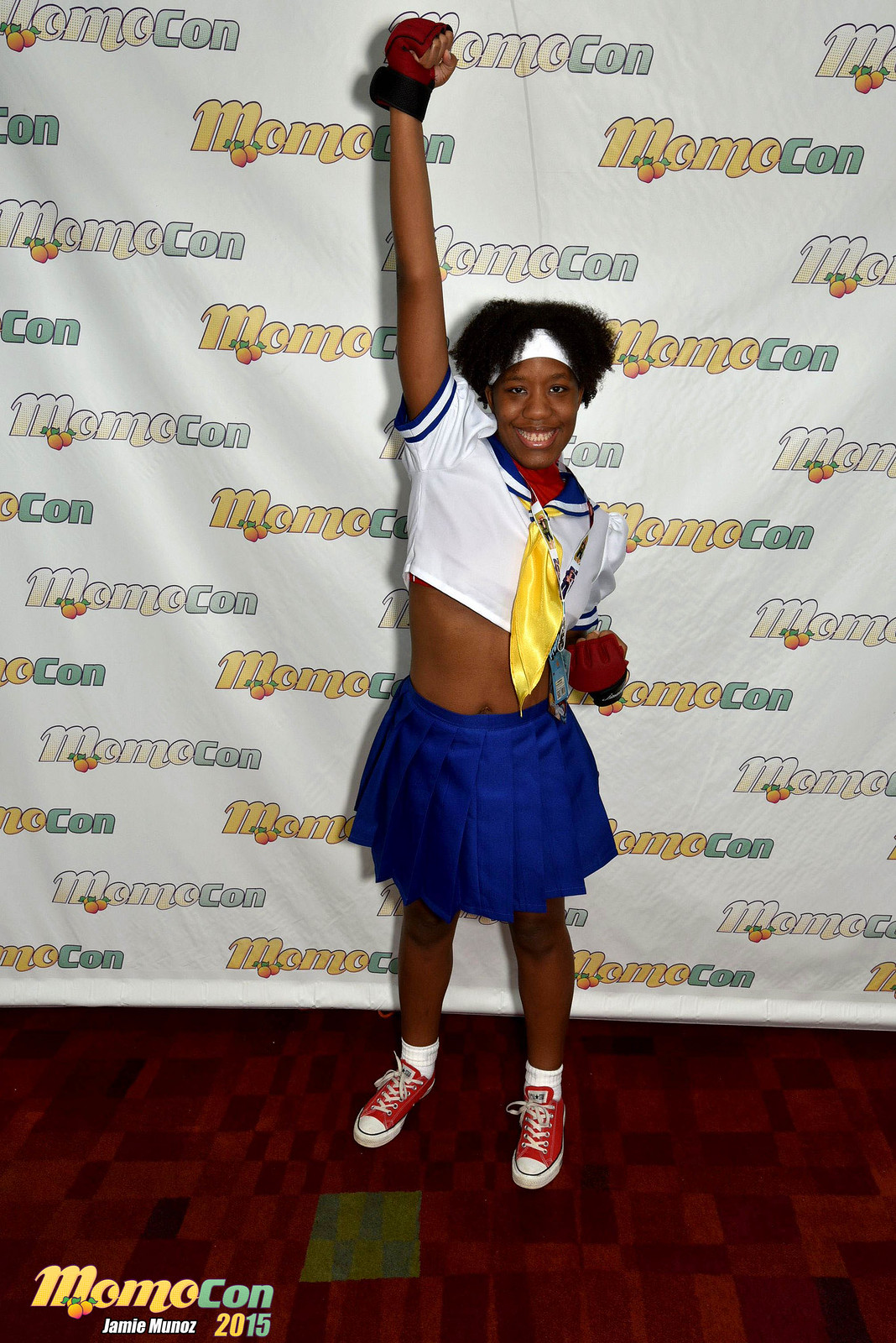A person dressed in a cosplay outfit reminiscent of Sailor Moon stands in the center of the photograph. They strike a dynamic pose with their right arm held high in a fist above their head and their left arm in a fist at their midriff. The individual has curly black hair and wears a white headband around their forehead. Their costume features a cropped white shirt with a blue and white sailor collar, blue trim around the arms, and a yellow tie. They pair this with a blue pleated skirt, red and white sneakers, and red gloves with thick black wristbands. The person stands on a red square carpet in front of a step-and-repeat banner with a white background. The banner displays the text "MomoCon" in peach, yellow, and blue, along with cartoon peaches. In the bottom left corner of the image, the text "Momo Khan, Jamie Munoz, 2015" is visible.